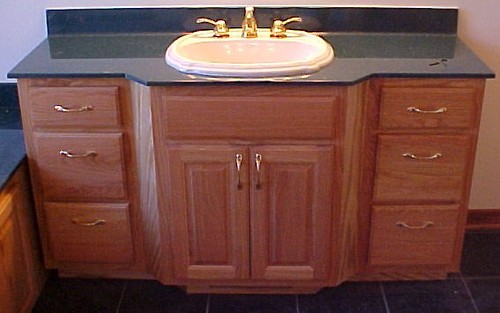This detailed indoor color photograph captures a newly installed vanity. The vanity base is composed of deep brown, wood-like material with a laminate finish. It features three columns of drawers on both the left and right sides. The central section projects slightly outward, accentuated by two vertical rectangular doors with dark metal or brass handles. The countertop is a striking deep blue marble, topped with a sleek white, oval, raised sink. The sink is complemented by a gold faucet with handles pointing horizontally to the left and right. 

The floor is covered in gray tile, adding a neutral backdrop to the colorful countertop. To the left of the vanity, a lower cabinet shares a similar bluish-gray countertop.

The background wall, coupled with a plastic baseboard, suggests the setting might be industrial or an office environment rather than a residential space. The entire setup looks pristine and unused, completely devoid of any objects or decorative items, underscoring its newly installed state. There are no visible words or text throughout the photograph.